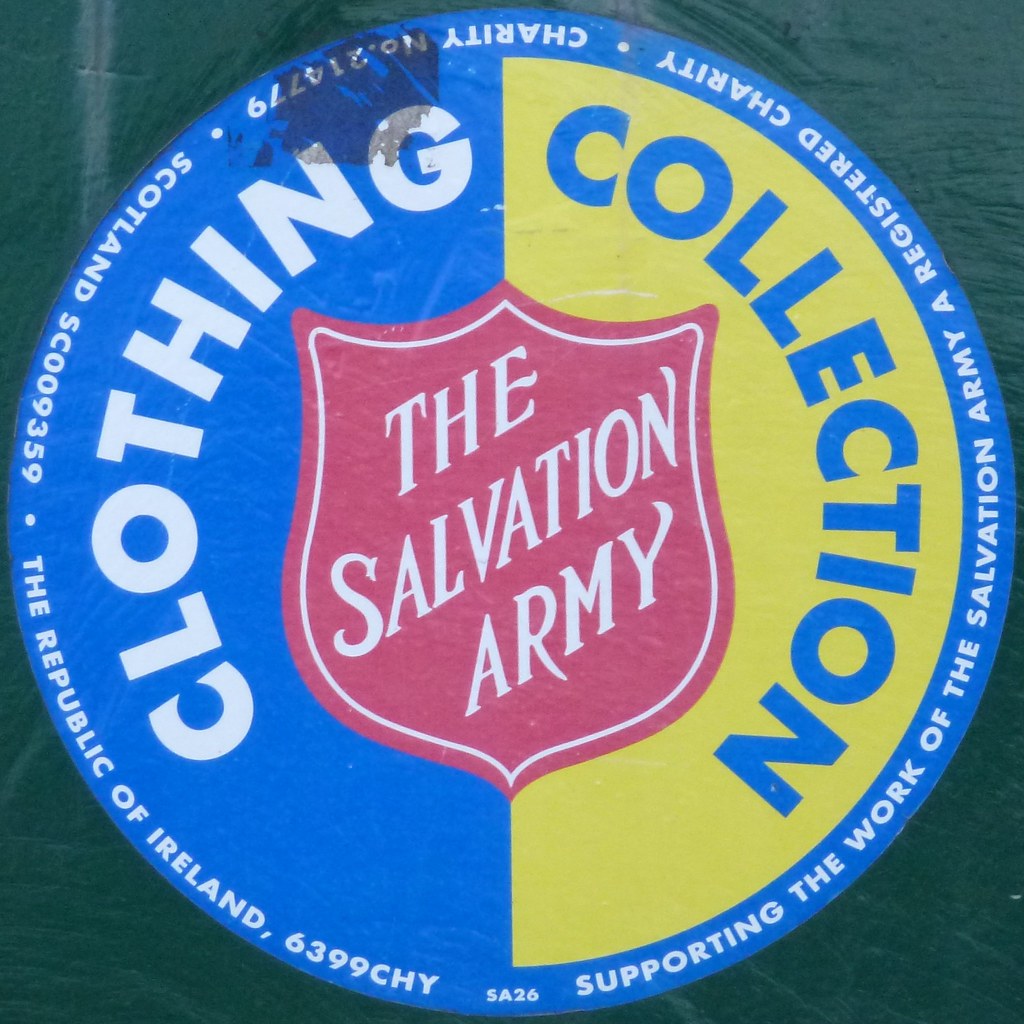In this image, we see a circular sign, likely a sticker or mounted poster, possibly designed for a business or charity collection point. The sign rests on a green background or wall. The central focus is a two-toned, blue and yellow circular banner. On the blue section, the word "Clothing" is prominently displayed, while "Collection" is written on the adjacent yellow section. In the middle of the circle, the iconic Salvation Army shield, vibrant in red with white text, prominently reads "The Salvation Army." Encircling the banner, additional text proclaims support for the work of The Salvation Army, a registered charity, with charity numbers listed as follows: 214779 for general reference, SC009359 for Scotland, and 6399CH for the Republic of Ireland.